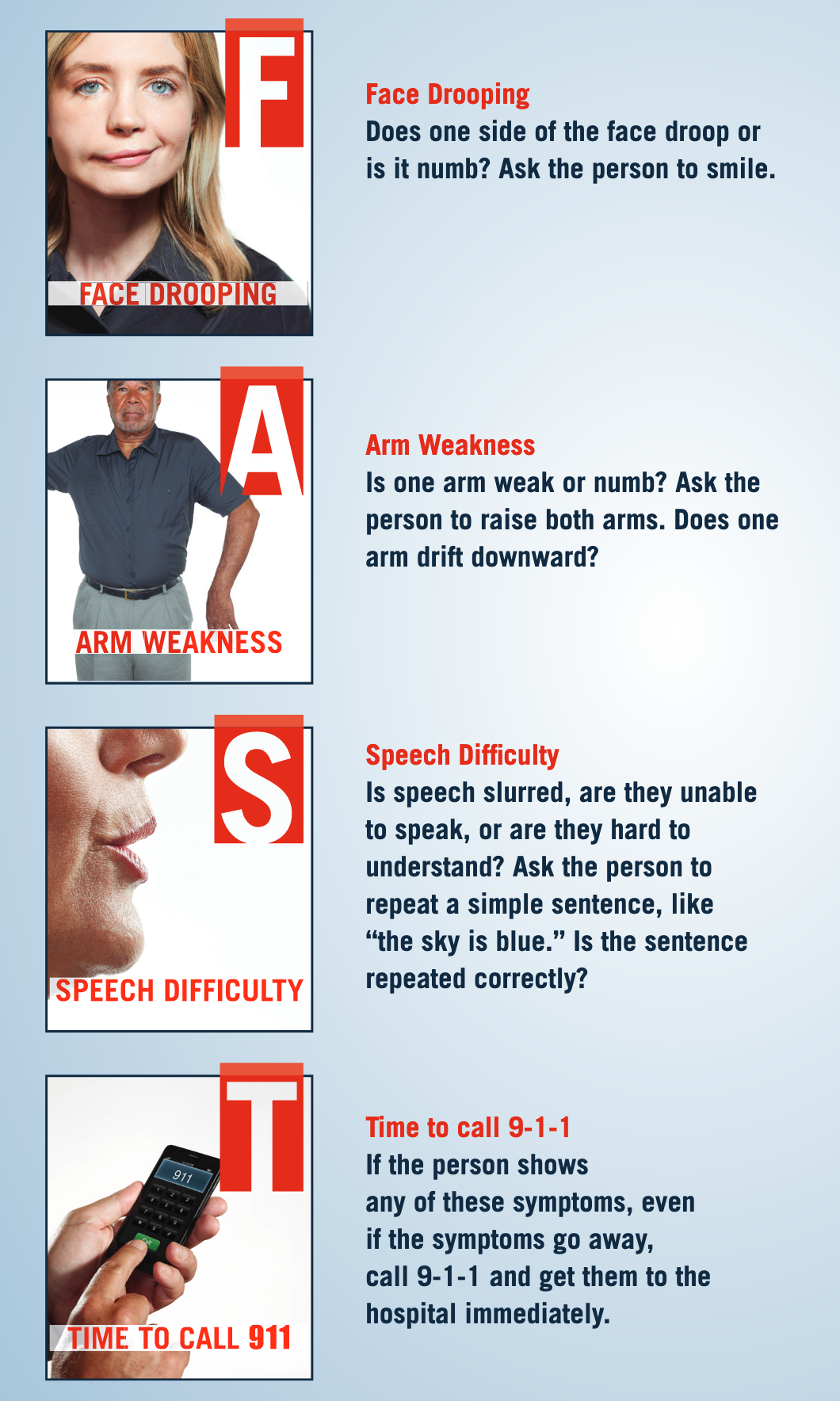This is a detailed medical poster designed to help recognize the signs of a stroke using the FAST mnemonic. The poster has a light blue background and features four key symptoms in both text and images, arranged vertically. On the left-hand side of the poster, each symptom is illustrated with images and labeled with large white letters with red outlines. 

At the top is "F" for face drooping, which shows a woman with one side of her smile sagging, indicating facial numbness or weakness. Next, "A" stands for arm weakness, depicted by a man struggling to lift his left arm. Following that, "S" represents speech difficulty and asks if the person’s speech is slurred, hard to understand, or if they are unable to speak. Finally, "T" reminds viewers that it’s time to call 911 if any of these symptoms are present.

On the right-hand side, the symptoms are clearly outlined with red headings: face drooping, arm weakness, speech difficulty, and time to call 911. Beneath each heading, blue text provides additional details on the symptoms and the essential action steps that should be taken. This poster serves as an essential guide for the early recognition of stroke symptoms, emphasizing the urgency of seeking immediate medical assistance.